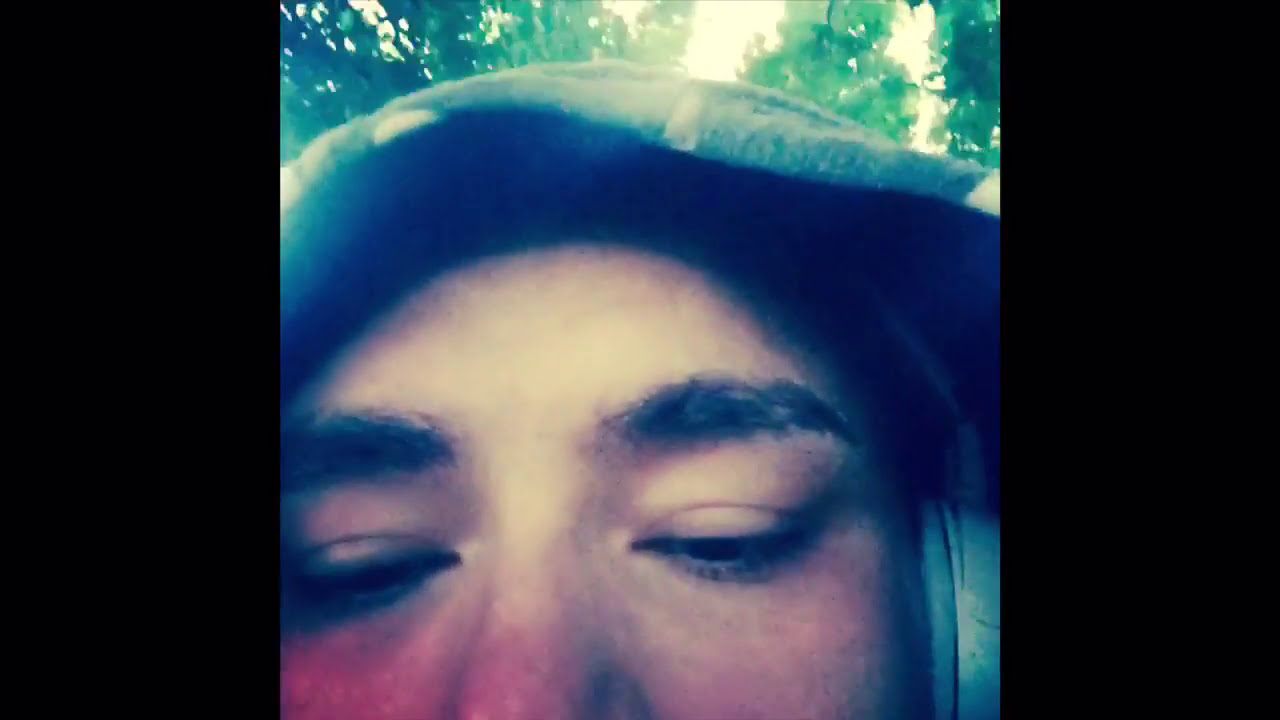This is an extreme close-up image of a man's face, occupying the central square portion of a horizontal rectangular frame with thick black bars on either side. The setting appears to be outdoors during the daytime, as indicated by the blurred green trees and sunlight peeking through in the yellowish background. The image, which has shades resembling almost but not quite a sepia tone, focuses on the man's eyes, bushy dark brows, and the top of his nose, while his head is slightly tilted downward. He has lightly tanned skin and dark brown facial hair. The man is wearing a hooded sweatshirt and gray over-the-ear headphones, which are partially visible under his hood on the right-hand side. The entire scene gives the impression of a still shot from a video or a selfie, which might have been taken using a phone.